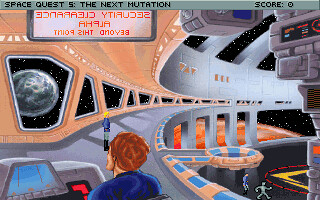A detailed screenshot from a computer game captures the immersive setting of a circular space station. The viewpoint is as if the observer is stationed on the upper level of the structure. A curved walkway extends to the right, drawing the eye into the depths of the station. Dominating the foreground is the back of a woman's head, positioned as she sits intently at a control console with multiple electronic display screens before her. Further down the curved walkway, another figure stands, possibly engaged in their own tasks. The scene extends to reveal a lower level, where another circular walkway hosts two indistinct figures. Framed by expansive windows, the backdrop of the space station is a starry black expanse of space, punctuated by the majestic presence of two visible planets. The juxtaposition of the detailed interior with the infinite universe outside creates an atmosphere that is both intimate and grand.